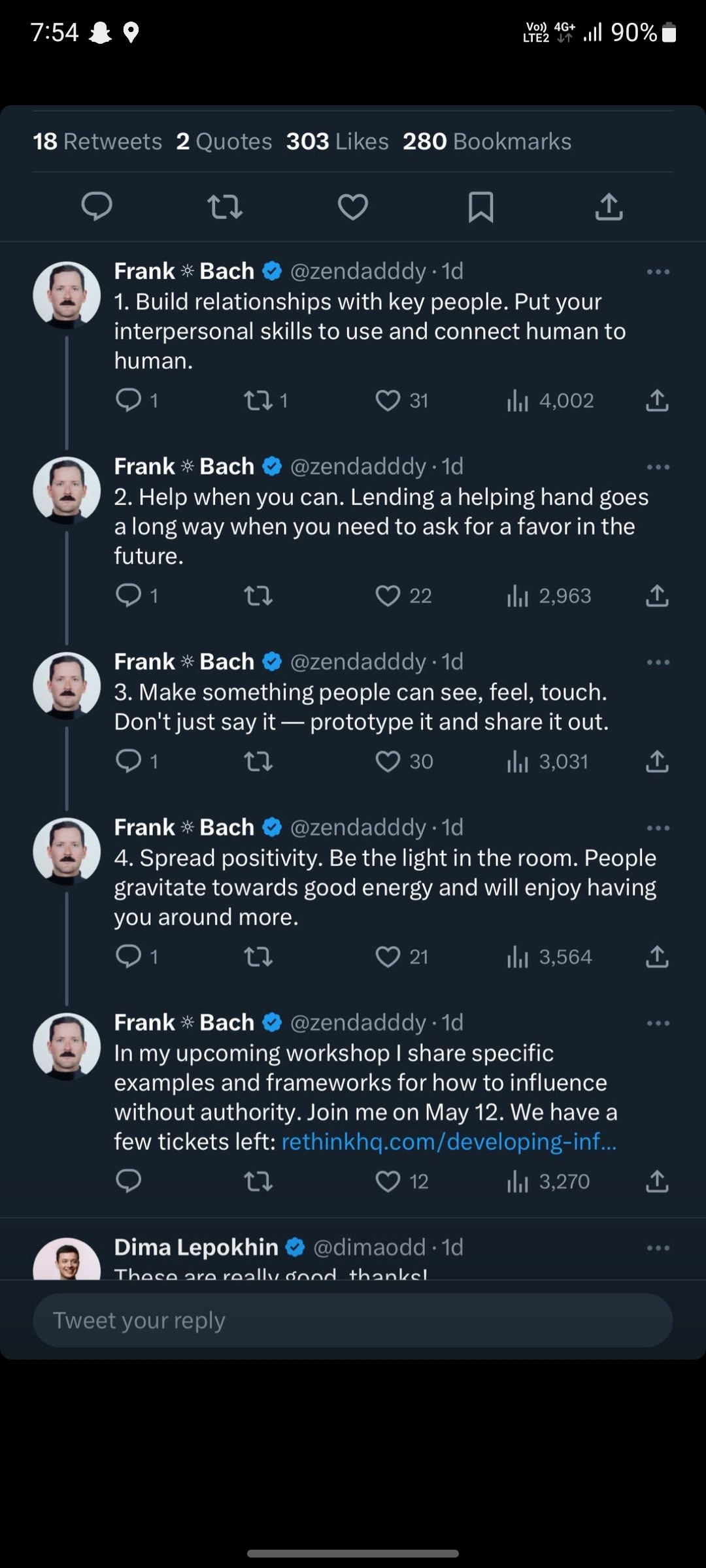**Caption:**

This social media interface image captures a tweet thread by Frank Bach, identifiable by his verified blue checkmark status. In the top left corner, there's a small ghost icon representing Snapchat, a location icon, and the battery indication, all in white. To the right, there's a display of "90%" battery, "VoLTE," "4G plus," alongside four signal bars in dark gray.

Within the tweet details at the bottom left, engagement metrics are shown in white and gray: 18 retweets, 2 quotes, 303 likes, and 280 bookmarks. There are standard icons for replies, retweets, likes, bookmarking, and a share arrow.

Frank Bach's tweet sequence includes valuable tips for interpersonal development:

1. **"Build relationships with key people"** - emphasizing the importance of human connection with one comment, 31 likes, and 4,002 views.

2. **"Help when you can"** - discussing the merits of offering help with one comment, 22 likes, and 2,963 views.

3. **"Make something people can see, feel, touch"** - advocating for prototyping with one comment, 30 likes, and 3,031 views.

4. **"Spread positivity"** - encouraging a positive demeanor with one comment, 22 likes, and 3,564 views.

Frank also mentions an upcoming workshop titled "Influence without Authority" with a URL link for more details, recording 12 likes and 3,270 views.

Dima Lepokhin, another verified individual, responds positively to Frank's tweets, leading into a "Tweet your reply" prompt in a gray banner below.

Overall, the profile picture consistently shows a man in his 30s with black hair, a black mustache, and a black turtleneck, slightly cropped within a white circular frame.